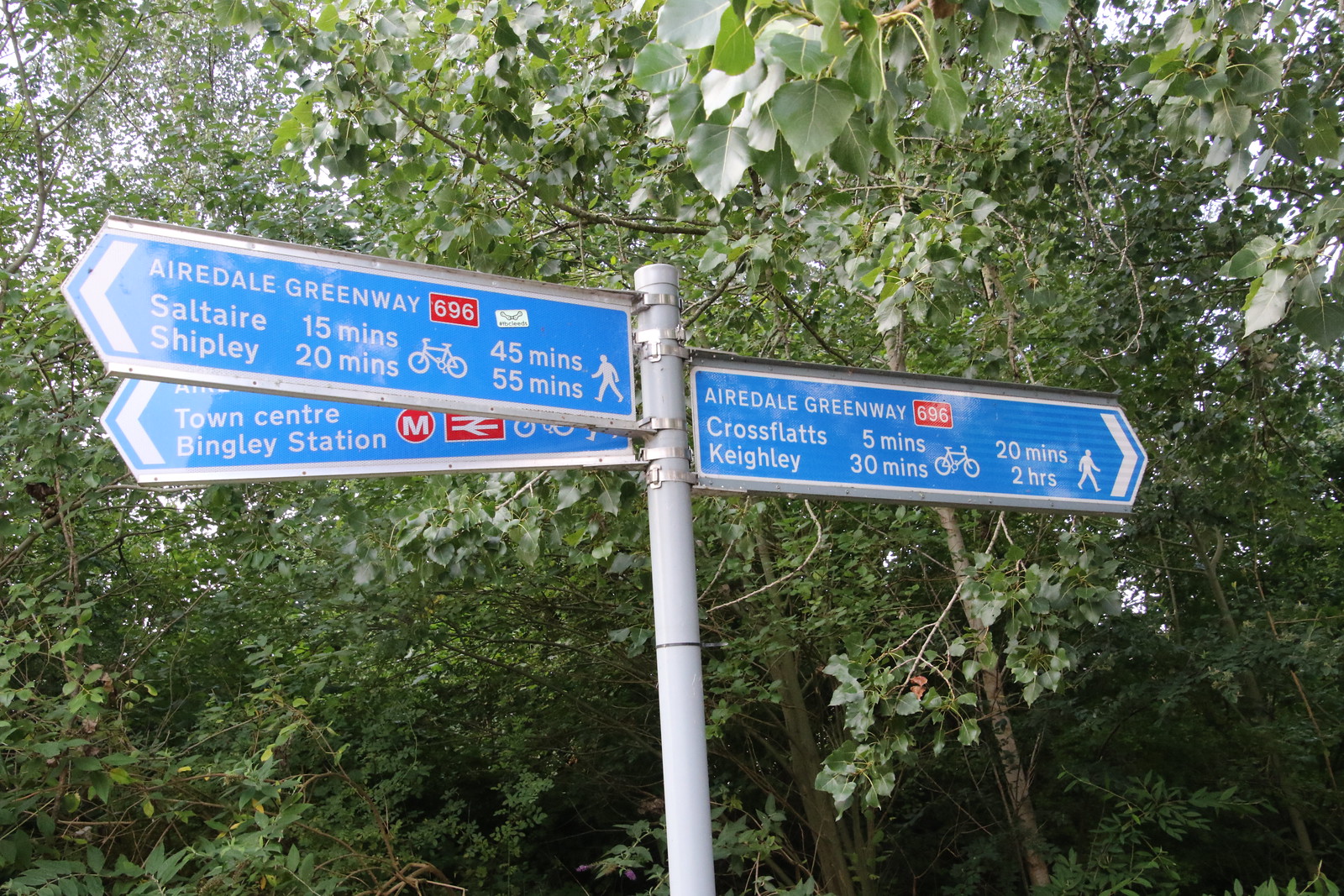The photograph captures an outdoor scene featuring a prominent signboard with three directional signs. The signs, blue with white text, are mounted on a silver pole. Each sign points in different directions: one to the right and two angled to the left. The right-pointing sign reads "Airedale Greenway, 696, Cross Flats, 5 minutes, Keegle, 30 minutes," along with bicycle and walking icons to denote travel times. The left-pointing signs include "Salterre, 15 minutes, Shipley, 20 minutes, Airedale Greenway, 696," and variants like "Town Center" and "Bingley Station." The background is lush with green trees and plants, and touches of sky peek through. This detailed signage likely serves pedestrians and cyclists navigating the Airedale Greenway pathway and its connecting routes.